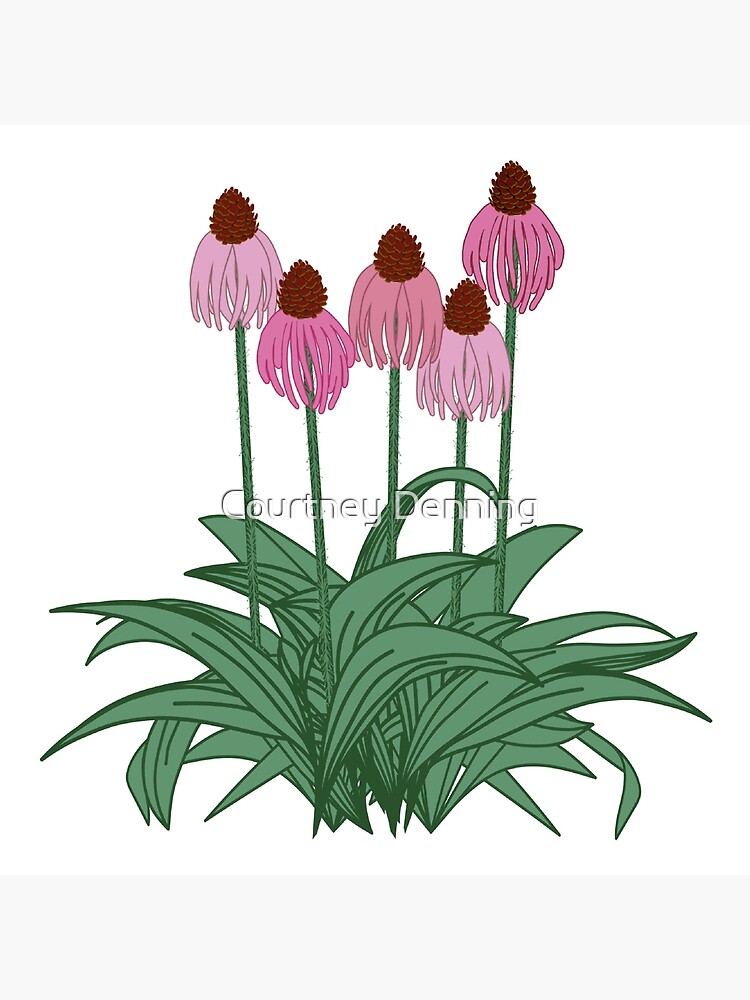This digital illustration features five pink and lavender flowers appearing wilted against a white background, with gray rectangles at the top and bottom. Each flower exhibits long, drooping petals reminiscent of flowing hair, and they are supported by green stems. The flower centers resemble small, dark red pine cones. The foliage comprises long, narrow, sharp-pointed leaves that interweave near the base of the stems. "Courtney Denning" is inscribed across the middle of the image, ensuring it cannot be copyrighted.